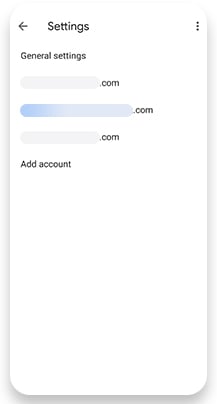The image depicts a settings menu, likely from a cell phone interface. The top of the screen features the title "Settings" along with a leftward-pointing arrow, which functions as a back button. Directly underneath, the header "General Settings" is visible. Beneath this header are several elongated rounded rectangles that appear empty but are placeholders for text input. These placeholders display "dot com" at the end. The first placeholder is grey, followed by a longer blue version, with another grey one at the bottom. At the very end, there is an option labeled "Add Account." The background is predominantly white, presenting a minimalistic and clean layout.